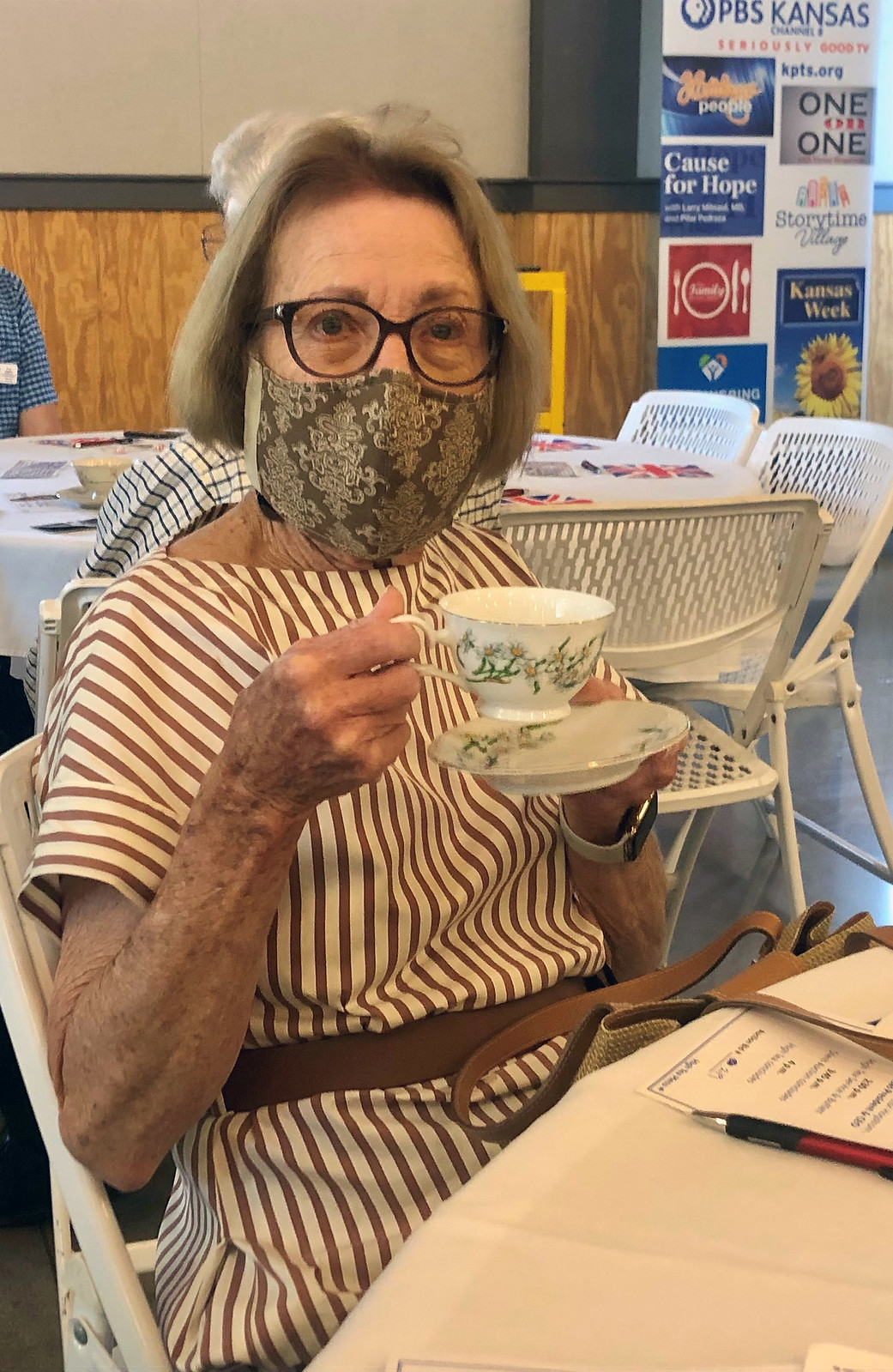An elderly woman, likely in her 70s or 80s, sits at a table in what appears to be a community event or cafeteria. She is seated on a white folding chair in front of a table adorned with a white tablecloth, with another similar setup visible in the background. The table in front of her has a piece of paper and a pen, and she has a purse in her lap. She is wearing a vertically striped dress in white and possibly reddish tones, paired with a face mask featuring a paisley pattern. In her hands, she holds a teacup and a saucer decorated with matching floral designs. The woman has short, shoulder-length dirty blonde hair and is wearing black, roundish glasses. Her aged skin shows some discoloration and wrinkles. Behind her, more elderly individuals are seated at another table, indicating that she is part of a larger gathering.